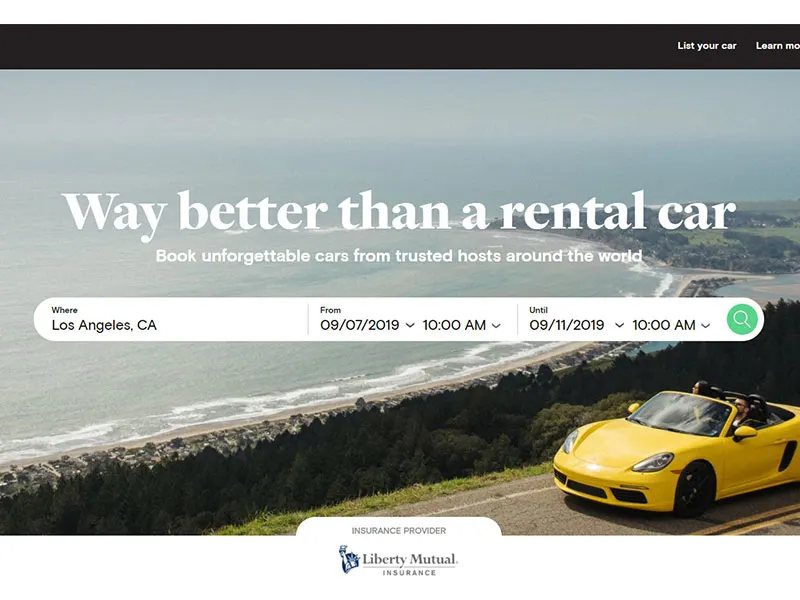This is a detailed screenshot of the Liberty Mutual website. At the top, there's a black horizontal strip featuring options such as "List Your Car" and "Learn More" on the right side. Just below this strip, in large white lettering, the text "Way Better than a Rental Car" is prominently displayed. Beneath this, a subheader reads, "Book unforgettable cars from trusted hosts around the world."

Below the text, there's a long oval search bar, indicating location and date input fields. The placeholder text in this bar reads: "Where: Los Angeles, California" with the dates "From: 09-07-2019, 10 AM" to "Until: 09-11-2019, 10 AM."

The background of the webpage features a scenic landscape divided into two halves. On the left side, there is a picturesque view of an ocean with a beach, bordered by a lush field of trees. On the right side, a vibrant yellow convertible sports car is depicted, with two people enjoying a ride.

At the bottom center of the image, the text "Insurance Provider" is clearly written. Below this, the name "Liberty Mutual Insurance" is displayed, accompanied by the iconic Statue of Liberty logo, specifically showcasing her head and torch-bearing arm.